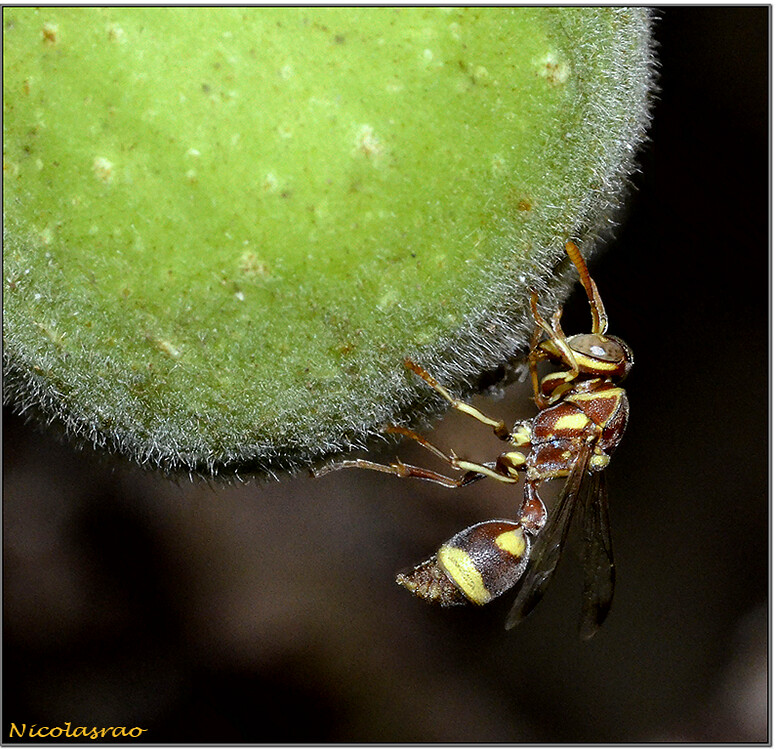This extremely close-up color photograph, likely taken outdoors, captures a highly detailed image of a wasp perched on a green, ball-shaped fruit-like object located in the upper left portion of the frame. The wasp, characterized by its yellow and black stripes and wings, sits with all its feet resting on the fruit, which is covered in tiny, whiskery white or silver hairs. The background is dark and blurred, creating a stark contrast that emphasizes the vivid details of the insect and the fruit. In the bottom right corner, yellow cursive text spells out "Nicolás Rao," presumably the photographer's name.